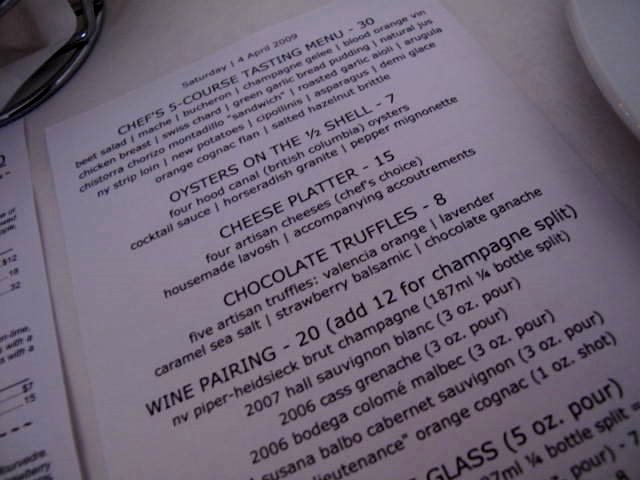A restaurant menu is delicately placed on a pristine white tablecloth, lending an air of elegance to the setting. On the table, a small round metal container, likely for napkins or condiments, adds a touch of modern utility. The menu itself is partially visible, with light gray paper and black text. At the top, the date "Saturday, April 4th, 2009" is prominently displayed. Highlighted on the menu is the chef’s five-course table menu offered at $30, featuring tantalizing choices like oysters on the half shell for $7, a cheese platter for $15, and chocolate truffles for $8. For beverages, a wine pairing is available for $20, with an option to add a champagne split for an additional $12. The menu details a variety of champagne options available, with the flexibility of combining champagne and wine for a unique dining experience.